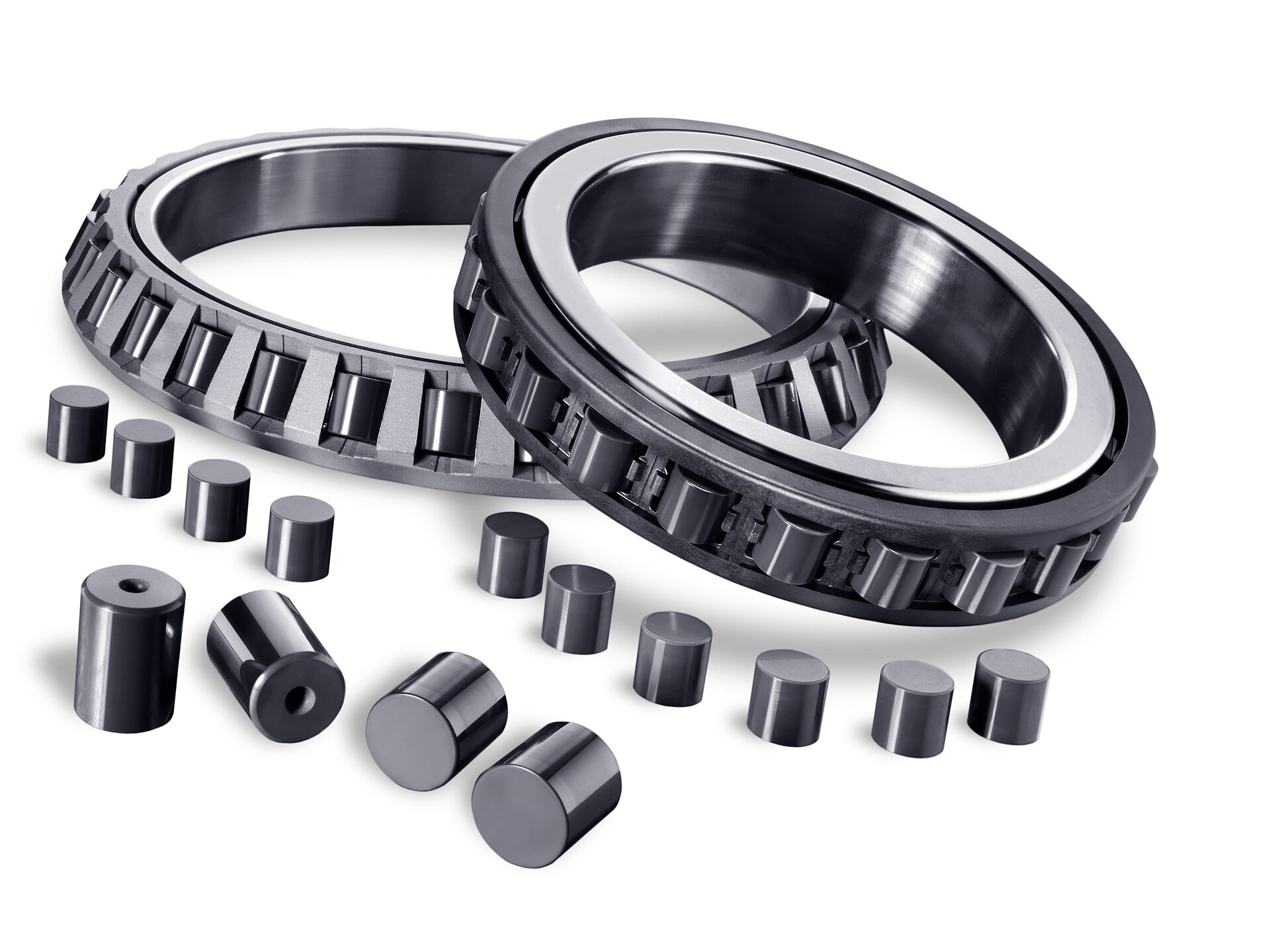The image showcases two metallic cylindrical rings, possibly automotive roller bearings, isolated against a bright white background. These ring bearings, predominantly grey and black, exhibit a shiny, reflective surface. Positioned below the rings are approximately 14 individual, thicker cylindrical parts that appear to be the rollers intended to fit on the exterior of the rings. The rings are stacked on top of each other, and the detailed close-up view highlights the metallic texture and precise engineering of these components, though the exact size of the rings remains unclear due to the lack of scale for perspective. The image is clear, well-lit, and devoid of any text or numbers, emphasizing the hardware components themselves.